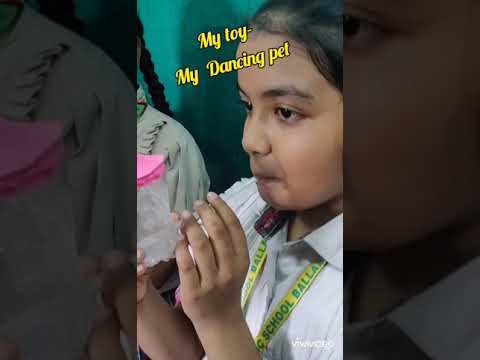The photograph depicts a young girl, likely of elementary school age with tan skin, possibly of Hispanic or Indian descent, standing beside another girl. The central image features the main girl with dark hair pulled back, wearing a white uniform with small shoulder flaps and a green band around her collar. Emphasized in the image is a clear semi-transparent glass container with a pink lid that she holds in her right hand, while her left hand hovers nearby as if to steady it. Her lips are puckered around a straw, suggesting she is drinking from the container.

The girl is positioned in front of a greenish-blue wall, and next to her, partially visible, is another child with black braided hair also dressed in a similar white uniform. Yellow text in the top center of the image reads "my toy" and "my dancing pet," which is slightly angled. The design is presented in a portrait mode, and the left and right sides of the picture are darkened, semi-transparent close-ups of the central image, mainly serving as a backdrop.